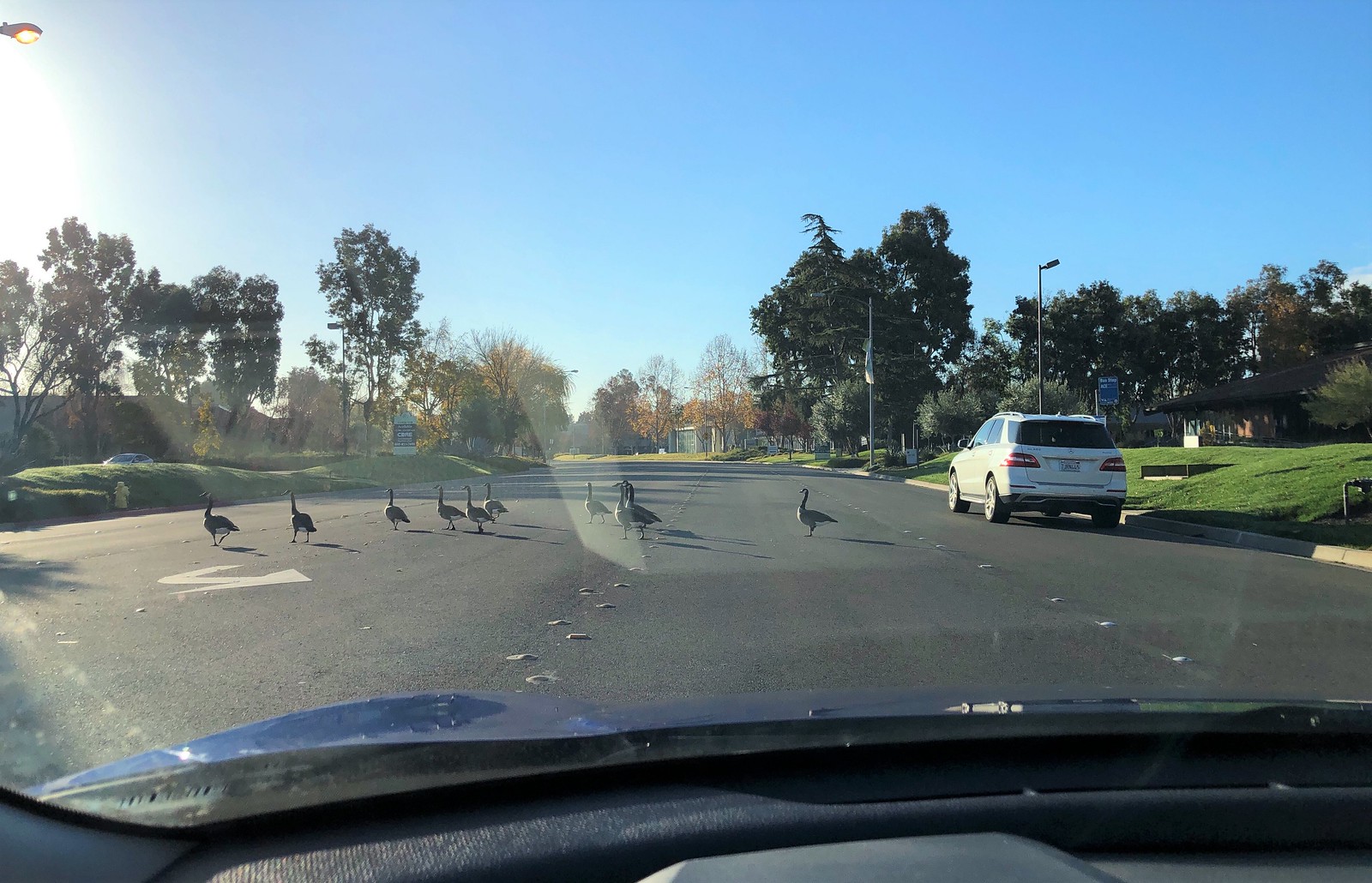The image captures the view from behind the steering wheel of a car driving down a scenic road on a bright, sunny day. The sky is a brilliant blue, with the sun visible in the upper left-hand corner, casting a warm glow over the scene. In the same corner, a street light extends into the frame. The street is flanked by sidewalks, lush green grass, and a scattering of trees. On the left side of the road, a wooden fence runs parallel, leading to a house visible in the distant background. To the right, there's a charming brick house with neatly manicured grass in front. A white car is parked along the curb. Dotted along the street are additional street lights and trees that add to the suburban charm. The focal point of the image is a small family of black ducks leisurely crossing the road, their presence adding a serene and whimsical touch to the moment. The car's dark gray windshield and part of the dashboard frame the lower portion of the image, anchoring the viewer in the driver's perspective.